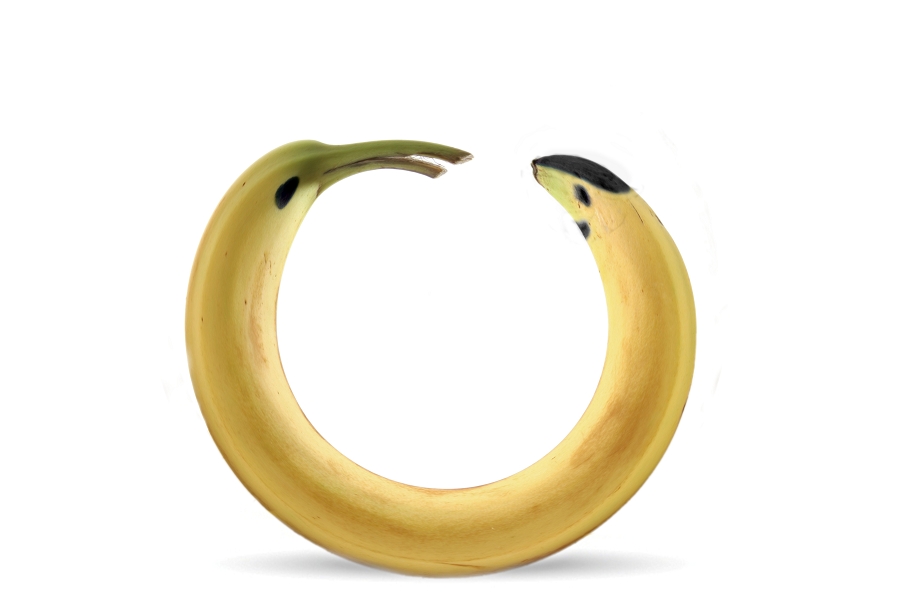The image features a uniquely distorted banana rendered against a white background. The banana forms an almost complete circle, resembling the letter "C" with its ends nearly touching but separated by a small gap at the top. The banana's peel is predominantly yellow but shows a few distinct color variations: the tail end on the right has black spots, while the stem end on the left is green with a black dot just below it. Additionally, the banana peel includes subtle brown tints along its length, enhancing the visual detail of the fruit.